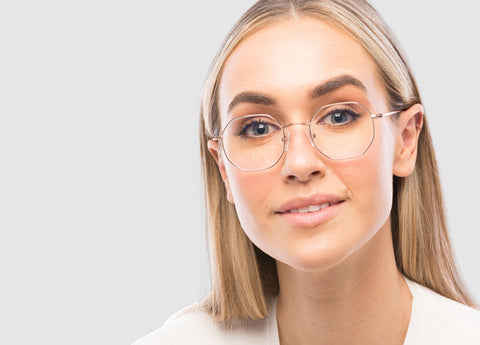In the image, a young woman appears against a light off-white to very light gray background, positioned slightly off-center to the right. She gazes directly at the camera with a slight smile, revealing her upper teeth. Her long, sandy blonde to dark brown hair, streaked with highlights, is tucked neatly behind her ears, accentuating her elegantly long neck. She wears round metal-framed glasses that hint at a professional demeanor, perhaps in the medical field. Her blue eyes, set under darker eyebrows, stand out against her clear, high forehead. She is adorned with pink lipstick and a small mole or flesh-colored bump just above her lip on the right side. The simplicity of her white top blends seamlessly with the unadorned background, enhancing the focus on her expressive, approachable face.